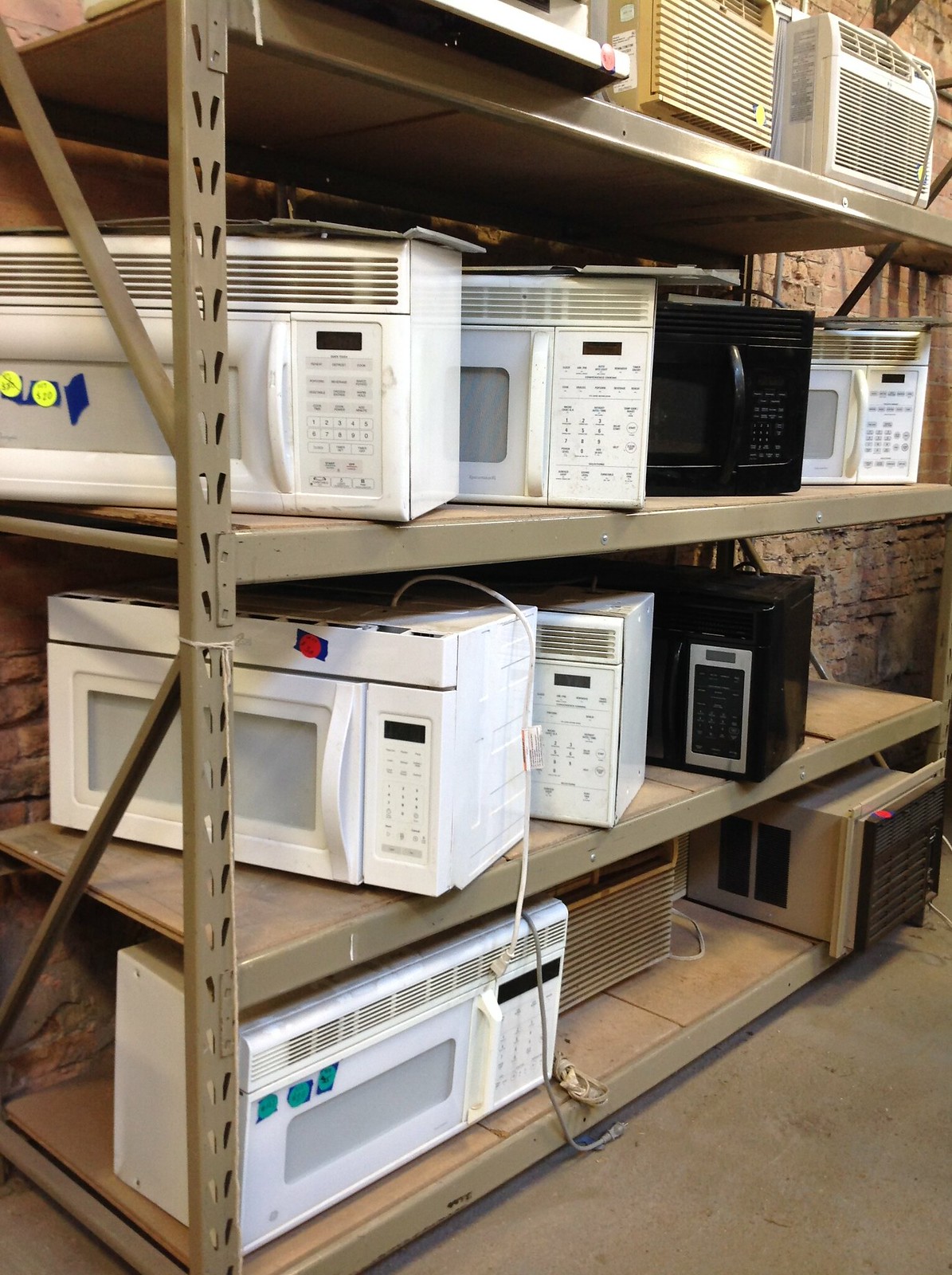The image shows a heavy metal display rack with four shelves, commonly found in a store or pawn shop. The shelves appear brownish-gray and hold a variety of used microwave ovens and window air conditioners, arranged in a somewhat stylish manner at angles. The top shelf features two window air conditioners—one off-white and the other white. The bottom three shelves contain both microwaves and air conditioners. Notably, the bottom shelf holds a white microwave and two air conditioners, while the second shelf features three microwaves (two white and one black), with cords notably draping down. The third shelf has four microwaves—three white and one black. The microwaves display various colored price stickers: teal, yellow, red, blue with red circles, and blue with green stickers, with one indicating a price of $20. These appliances look heavily used, some showing signs of wear on their cords, and none appear to be plugged in or operational. The positioning of the photograph is angled, allowing a clear view of the control panels on the microwaves.